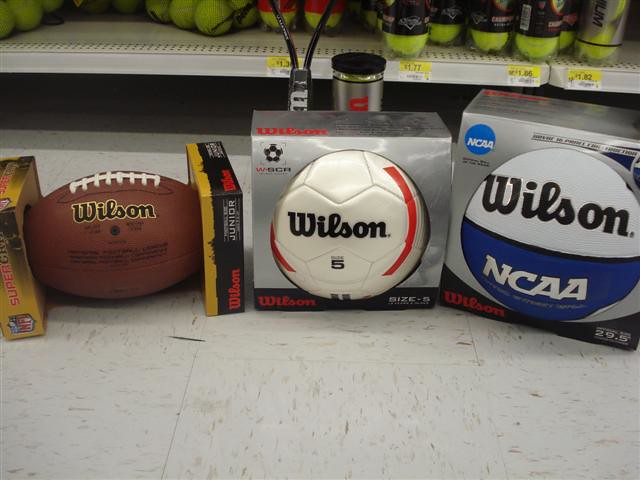In a bustling sports shop, the image captures the bottom section of a white shelving unit filled with neatly arranged tennis balls, both stacked upright in cylindrical containers and laid flat. The shelf displays standard green-yellow tennis balls in assorted packaging, with price tags clearly visible along the edge.

In front of this shelving, three sports balls, still in their original packaging, dominate the scene. Positioned on a slightly dirty, speckled white linoleum floor, the balls are laid out from left to right. The first ball is a Wilson Junior American football, donning a classic brown leather with white stitching and a large Wilson logo in black with gold trim, partially obscured by its two-sided yellow-black packaging. 

Next is a Wilson size 5 soccer ball, primarily white with red stripes, encased in a silver cardboard box that prominently displays the Wilson logo. 

To the right is a Wilson NCAA basketball, its top half white and bottom half dark blue, with the Wilson branding in black on the white and NCAA in bold white letters on the blue. It, too, is nestled in a similar silver box.

Partially visible behind these balls are additional sporting goods: a can of tennis balls with a silver label and red font and a tennis racket resting against the shelf, adding to the vibrant assortment of sports equipment in this aisle.